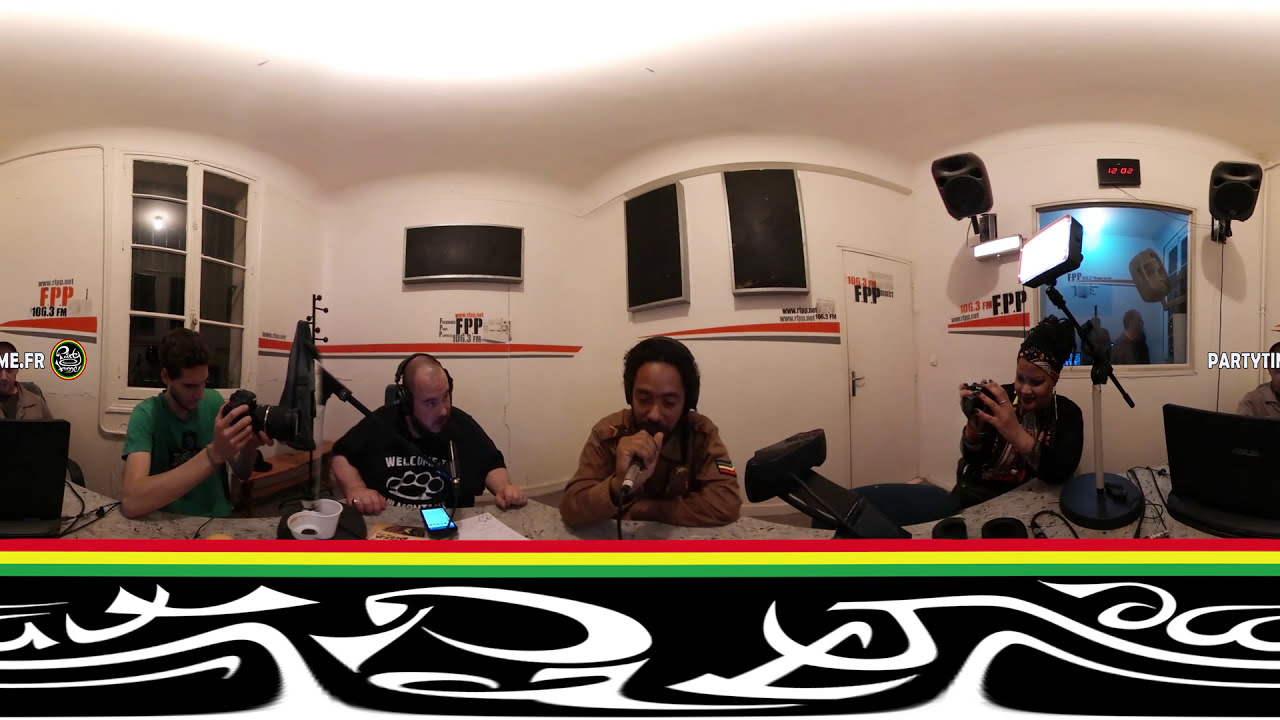In the image, we see a bustling recording studio, possibly used for a radio show or podcast. Five people are gathered around a large, speckled gray table within a small, white room. At the center of attention is an African American man in a tan shirt, holding a microphone in his right hand. To his left is a balding Caucasian man in a black shirt, wearing headphones and also having a microphone on a stand.

The setup is busy with various recording equipment, including cameras wielded by a female and another man on the far left, both aiming their lenses at the man in the center. The background features windows and doors, providing a glimpse into other parts of the studio, and the walls are adorned with speakers, lights, and other equipment.

Colors in the image are vivid, with red, yellow, and green stripes running across the bottom, reminiscent of a Rastafarian banner. Below these stripes, there's a black section with white, swirling patterns. The image gives a panoramic view, resulting in some distortion but capturing the essence of a lively, indoor recording environment.